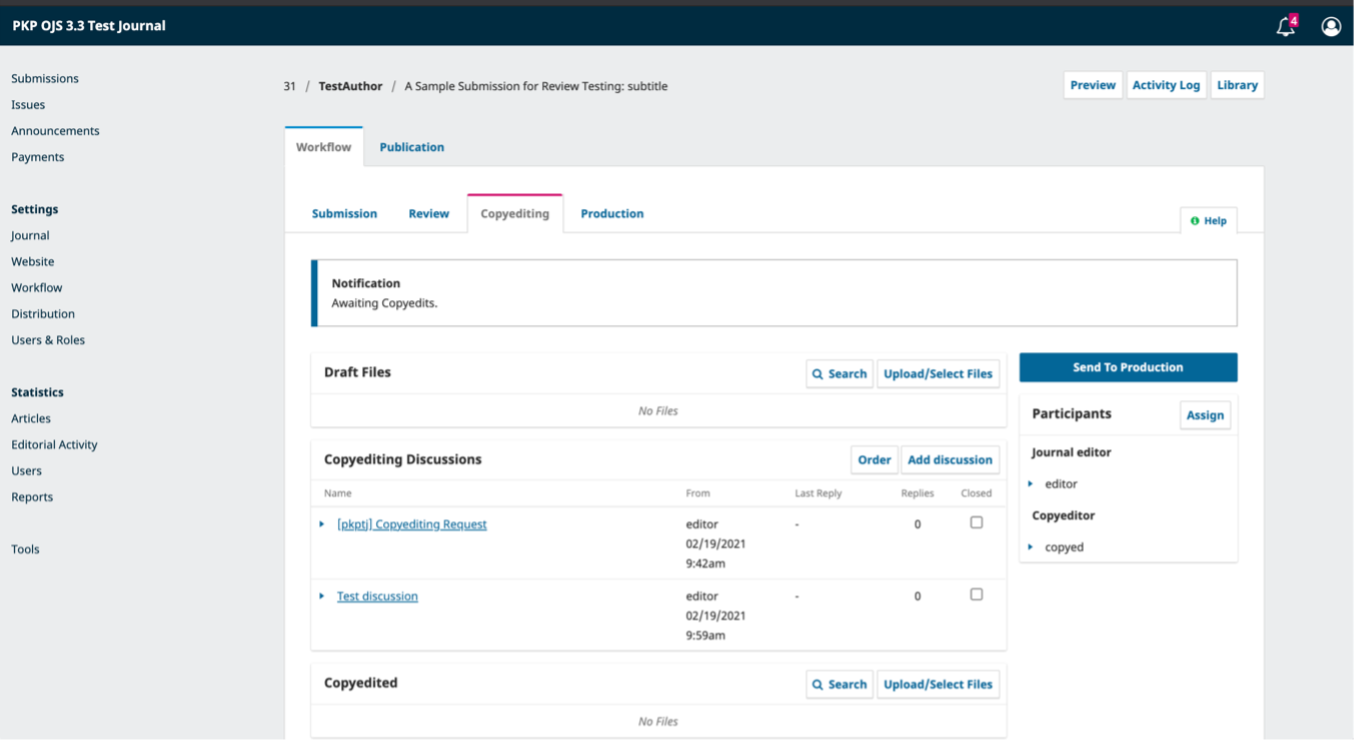The top section of this web page features a dark blue background. On the left-hand side, the title "PKB OJS 3.3 Test Journal" is displayed in white text. On the right side, there's a white outline of a bell icon and a magenta-colored rectangle with the number "4" in white. Adjacent to this is a white circle containing a white silhouette of a person.

Beneath the header, the background shifts to a gray color. The left-hand side consists of a vertically arranged menu in dark blue text that includes the following options: Submissions, Issues, Payments, Payment Settings, Journals, Website, Workflow, Distribution, Users & Roles, Statistics, Articles, Editorial Activity, Users, Reports, and Tools.

At the top section of this gray background area, there is a black text line that reads "31/test author/sample submission for review testing...subtitle". Below this line, three white boxes outlined in gray are labeled "Preview," "Activity," and "Library," with blue text.

At the bottom, there are two tabs. The first tab is white with gray text and a blue underline labeled "Workflow," while the second tab has a gray background with blue text labeled "Publication". Inside the "Workflow" tab, there are four additional sub-tabs. The first two sub-tabs are teal and labeled "Submission" and "Review". The third sub-tab is gray with a magenta underline, labeled "Copyediting". The fourth sub-tab is teal, labeled "Production". Currently, the "Copyediting" tab is open.

In the "Copyediting" section, black text indicates a notification: "Awaiting Copyedit." The status is "Draft," and there are no files in the copyedit. A discussion thread is shown with black text, noting two replies: "From Last Reply" and "Reply Close". The thread was edited on "02/19/2021 at 9:42 AM" and "02/19/2021 at 9:59 AM."